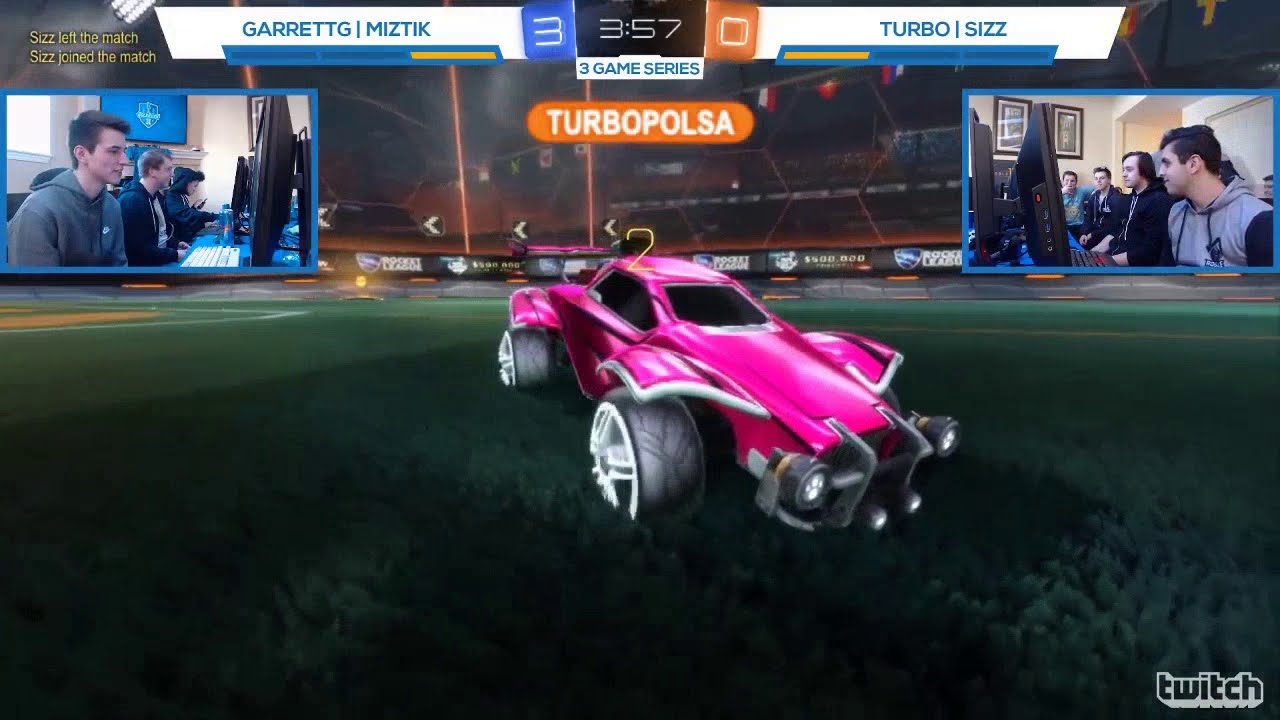This image is a screen capture from a video game, prominently featuring a bright pink, retro-looking race car with bold red highlights, large black tires, and silver wheels, parked on a field of dark green grass. The setting is a large, nighttime stadium with multiple tiers of empty stands, adorned with advertisements reminiscent of those seen around a soccer field. Bright stadium lights illuminate the scene, enhancing the vibrant atmosphere.

At the top of the image, game-related information is displayed. In blue and white text, the scoreboard reads "Garagi Mystic 3 - 3:57 - 3 Games Series - 0 TurboSys." In an orange highlight, it mentions "TurboPulsa." Additionally, there's text indicating game events, such as "Ciz left the match" and "Ciz joined the match." Below this, in smaller sections, are photographic images of the game participants. On the top left side, three individuals are seen intently looking at large monitors, with mixed expressions of concentration and smiles. Similarly, on the top right, four individuals are also focused on their screens.

At the bottom of the image, the Twitch logo is prominently displayed, indicating that the scene is being streamed live on this popular platform.